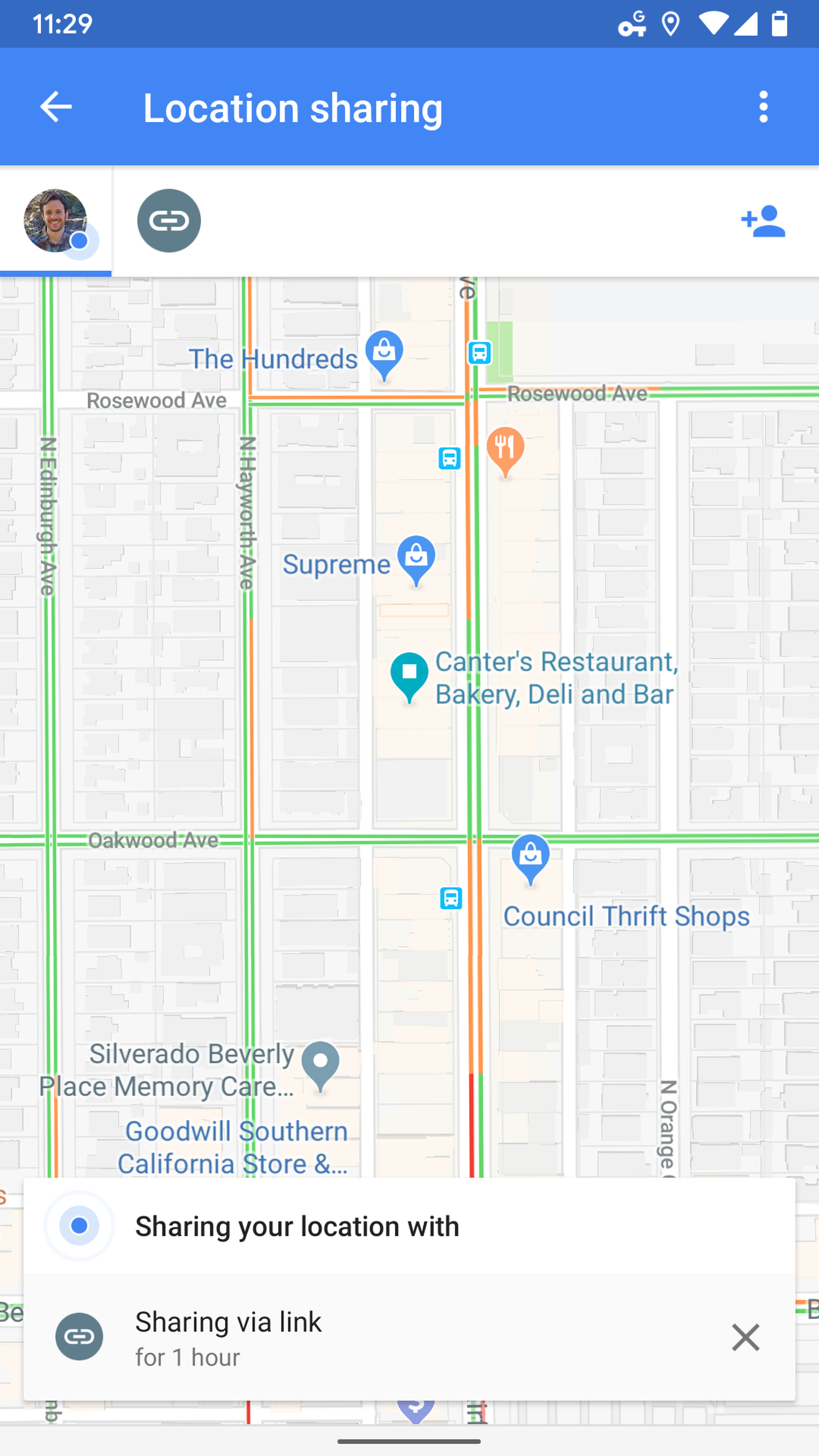This image depicts a location-sharing interface on a mobile phone. At the top, there's a thin blue bar displaying the time "11:29" along with the typical phone icons on the right side. Directly below, a lighter blue bar contains white text that reads "Location Sharing," accompanied by a white arrow pointing left.

Beneath this is a white bar featuring a user icon and two additional icons. The majority of the image is dedicated to a detailed map that showcases several notable locations. Among these are "The Hundreds" at the top, "Supreme," "Cantor's Restaurant, Bakery, Deli, and Bar," "Council's Thrift Shops," "Silverado Beverly Place Memory Care," and "Goodwill Southern California Store."

Overlaid on the map is a white box presenting two options. The top line, in bold black text, states "Sharing your location with," while underneath it is the phrase "Sharing via link for one hour." To the right of this text is an X, presumably for closing the overlay.